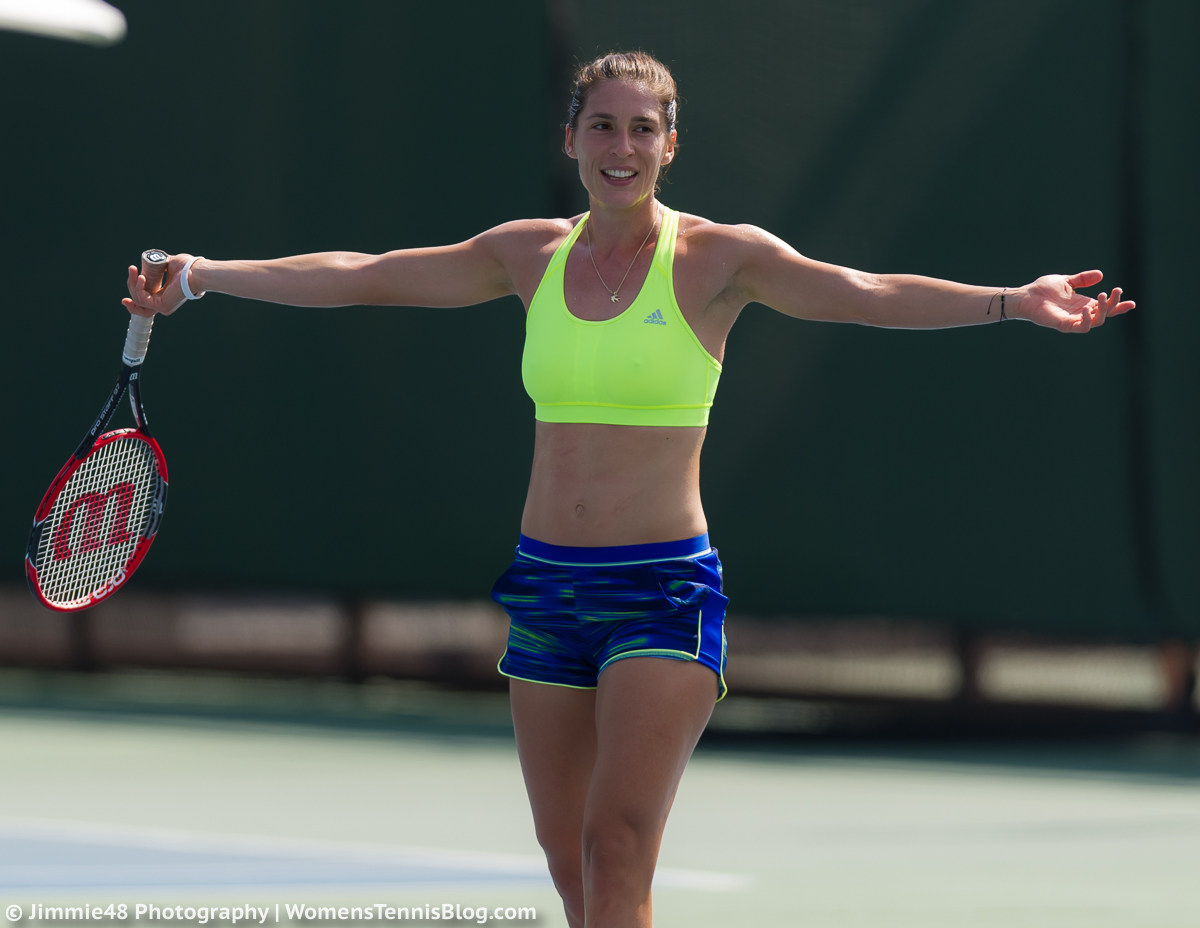In this vibrant photograph taken by Jimmy48 Photography for womenstennisblog.com, a young female tennis player, Maria Petrovic, stands prominently in the center. Maria, who appears to be around 10 years old, is captured in an outdoor tennis area, wearing very short blue and yellow striped shorts paired with a fluorescent yellow sports bra from Adidas. Her long hair is tied back in a ponytail, and she sports a white wristband on her right wrist along with a string bracelet or possible black tattoo on her left wrist. Maria's arms are outstretched with her palms facing up, her right hand grasping a red, black, and white Wilson tennis racket pointed downward. She is looking off to the right side of the image, smiling with an open mouth, exuding happiness as she gazes intensely at something out of frame. The backdrop features a blurry tennis court with hints of green and blue lines, enhancing the focus on Maria. The bottom corner of the photo contains a white text watermark that reads "copyright jimmy48photographywomenstennisblog.com".